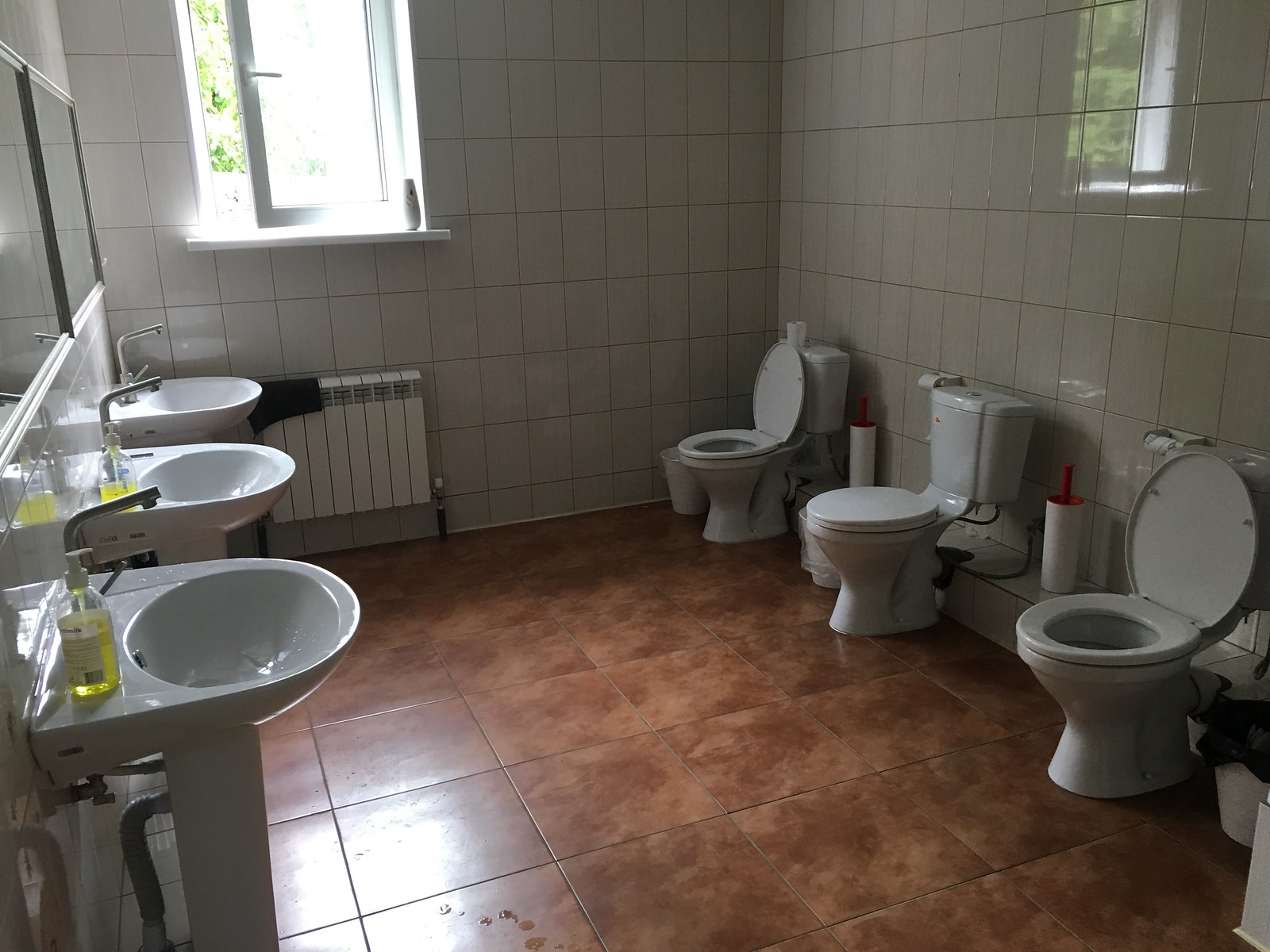This photograph showcases a meticulously detailed bathroom. The floor is adorned with large brown tiles, while the walls are covered in shiny white tiles that add to the room's brightness. On one side of the room, there are three white porcelain toilets, each equipped with a small cistern. The outer toilets have their lids up, while the central one has its lid down. Behind each toilet, there are toilet paper dispensers, accompanied by small bins and wall-mounted toilet brushes with red handles. Between the toilets, there is a roll of paper towels. Opposite the toilets are three white porcelain sinks, each adorned with yellow liquid soap bottles on the front two sinks. Above these sinks is a large white-framed mirror. On the back wall, there is a white radiator heater with a piece of black fabric on top. Above the radiator is an open casement window with a white sill, which provides a glimpse of vibrant greenery outside, adding a touch of nature to the pristine environment inside.